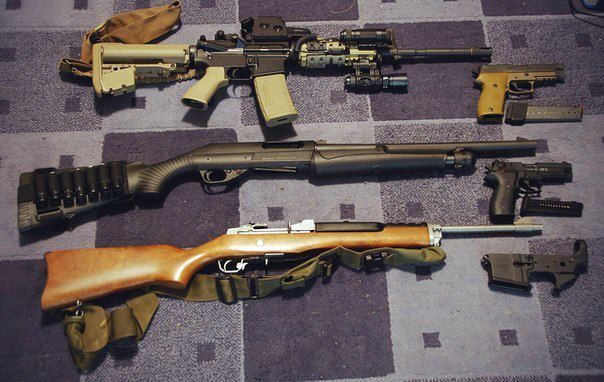The image showcases a lineup of firearms meticulously arranged on a textured gray and black checked carpet, which appears slightly worn and dirty. From top to bottom, the collection comprises six guns varying in type and size. At the top of the lineup is a machine gun, notable for its beige coloration and numerous components, including a prominent magazine that suggests military use. Beneath it, there's a shotgun with dark gray gunmetal and black accents, outfitted with a brownish-green strap and shotgun shells attached, ready for loading. Following this is an AK-47, featuring a green grip and a brownish-bronze steel body and barrel. Further down, a light tan wooden shotgun with a stainless steel barrel stands out with its rustic look, accompanied by a strap. On the far right, two smaller handguns in black and light yellow-gray tones rest with their clips displayed beside them. The firearms range in shades of gray, beige, black, and brown, creating a visually diverse yet cohesive armament display.